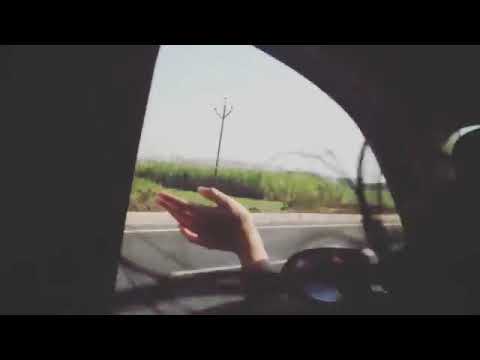This grainy and retro-styled photograph captures a moment from inside a vehicle, looking out through a triangular, beveled window. The scene is dominated by a Caucasian hand extended out of the window, with fingers slightly open as if catching the breeze. Long hair wisps into the frame, adding to the sense of movement and freedom. The interior of the car is cloaked in darkness, making the outside scene the primary focus. Beyond the window, there's a paved road leading to a shoulder area, adjacent to what appears to be a field of green farmland or possibly corn. A single power pole stands upright in the field under a light gray, blue sky, subtly emphasizing the rural and open landscape.